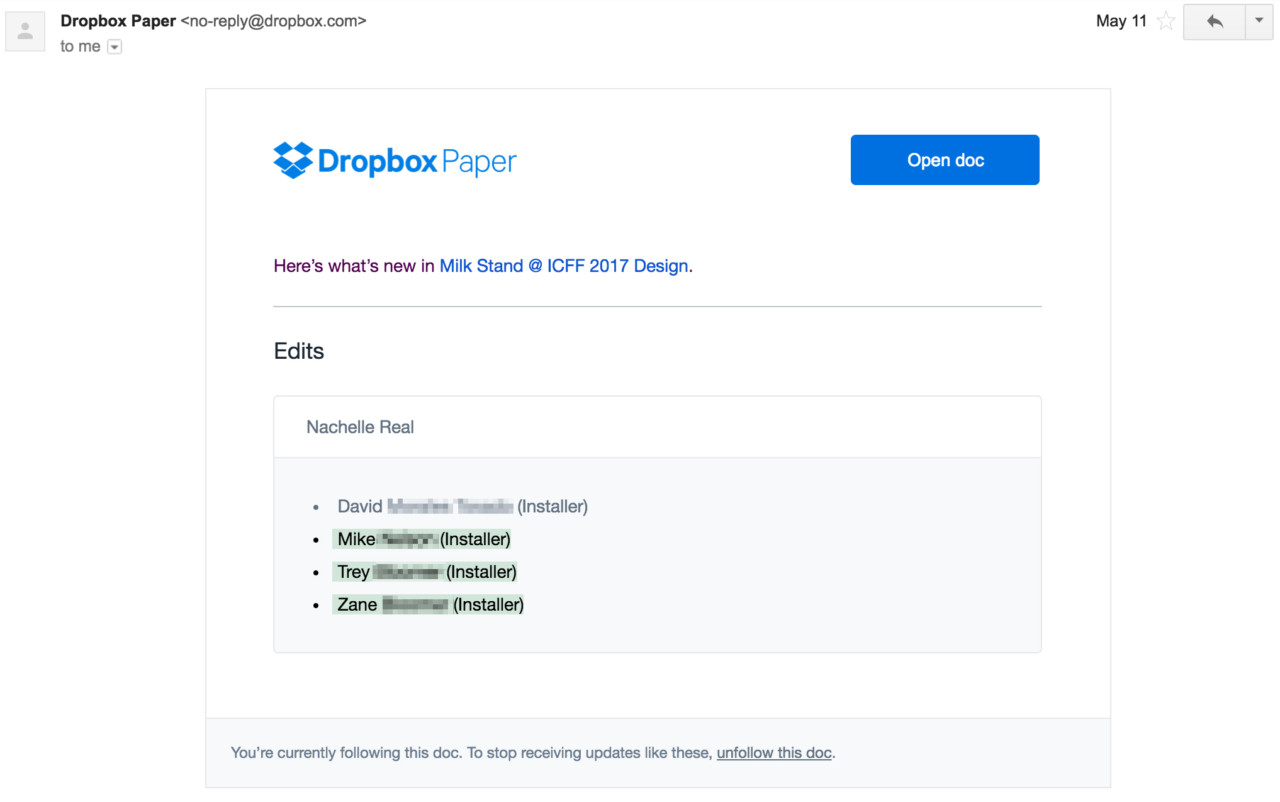The image displays the body of an email sent from Dropbox Paper. At the very top-left corner, there's a small gray box featuring an animated head and shoulders icon. Next to this icon, "Dropbox Paper" is displayed in bold black print, followed by the sender's email address, no-reply@dropbox.com. Beneath this, it indicates the recipient as "me" with a drop-down arrow box.

On the top-right side of the image, the email's date, May 11th, is shown along with an outlined star and a drop-down box featuring the "Reply All" arrow.

The main body of the email occupies a white square. Within it, the Dropbox Paper logo, characterized by a blue open cardboard box icon, is placed to the left of the word "Dropbox." Adjacent to this logo is a blue button labeled "Open Doc" in white font. Below this button, the text reads: "Here's what's new in Milk Stand at ICFF 2017 design." A line separates this section from the rest of the email content.

Following this line, the section titled "Edits" begins. It features a rectangular box with a white header labeled "Michelle Real." The body of the box is a light gray color and contains four bullet points with names: David, Mike, Trey, and Zane. The last names are blurred out, and after each name, the term "(Installer)" is included in parentheses. Additionally, the names Mike, Trey, and Zane are highlighted in light green.

At the very bottom of the image, there is a small gray box spanning the width of the email. It states: "You’re currently following this doc. To stop receiving updates like these, unfollow this doc," with "unfollow this doc" underlined and appearing as a clickable link.